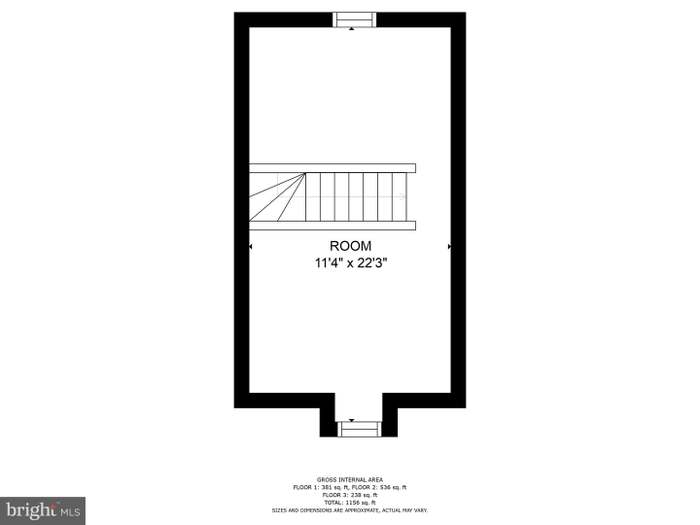This image is a detailed blueprint of a rectangular room, bordered by a thick black outline. The room dimensions are clearly marked, measuring 11 feet 4 inches by 22 feet 3 inches. The blueprint shows both horizontal and vertical lines that further define the structure. There are several entrances and exits, including a doorway at the top and another at the bottom, alongside depicted steps in the center leading either up or down. 

Additional details indicate the gross internal areas for three floors: Floor 1 is 381 square feet, Floor 2 is 538 square feet, and Floor 3 is 238 square feet, summing up to a total of 1,156 square feet. These measurements and conversions are noted to be approximate and subject to variation. All text is displayed in capital letters, and at the bottom right corner, there is a gray rectangular background with the text "Bright MLS," suggesting that Bright may be an architectural or construction firm responsible for the design. The room is illustrated as empty, showcasing its unadorned structure and layout.